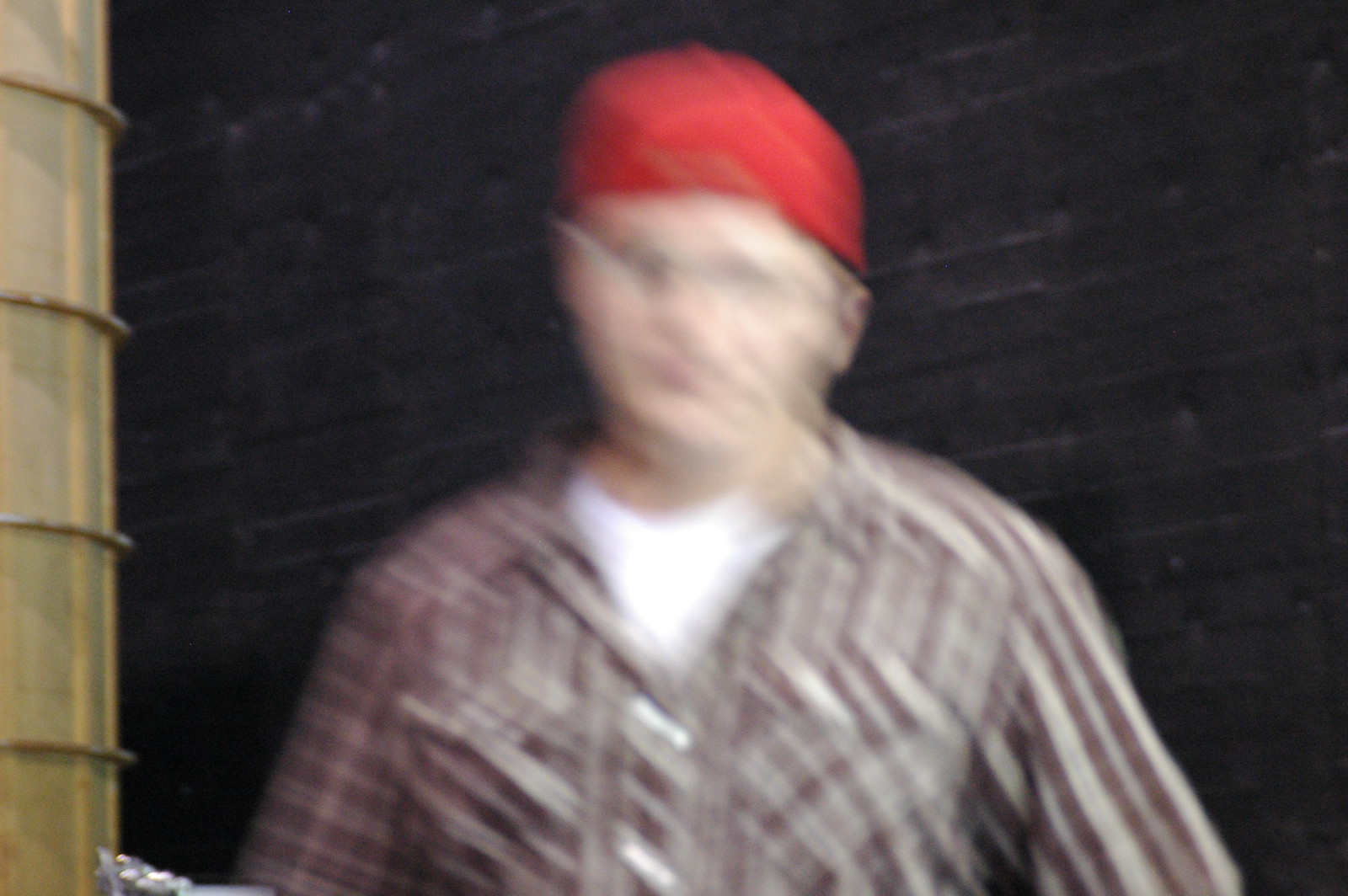This image captures a scene in motion, resulting in an extremely blurry depiction of a man outside. Despite the haziness, it's discernible that he is dressed in a red cap and layered in a white undershirt beneath a purple and white striped flannel shirt. The man appears to be Caucasian and is standing in front of a dark, black brick wall. To the left of the frame, there is a faded beige or yellow pole with four evenly spaced circular bars around its circumference. In the bottom left corner, part of a silver camera or cell phone device is visible, likely explaining the photograph's blurred quality.